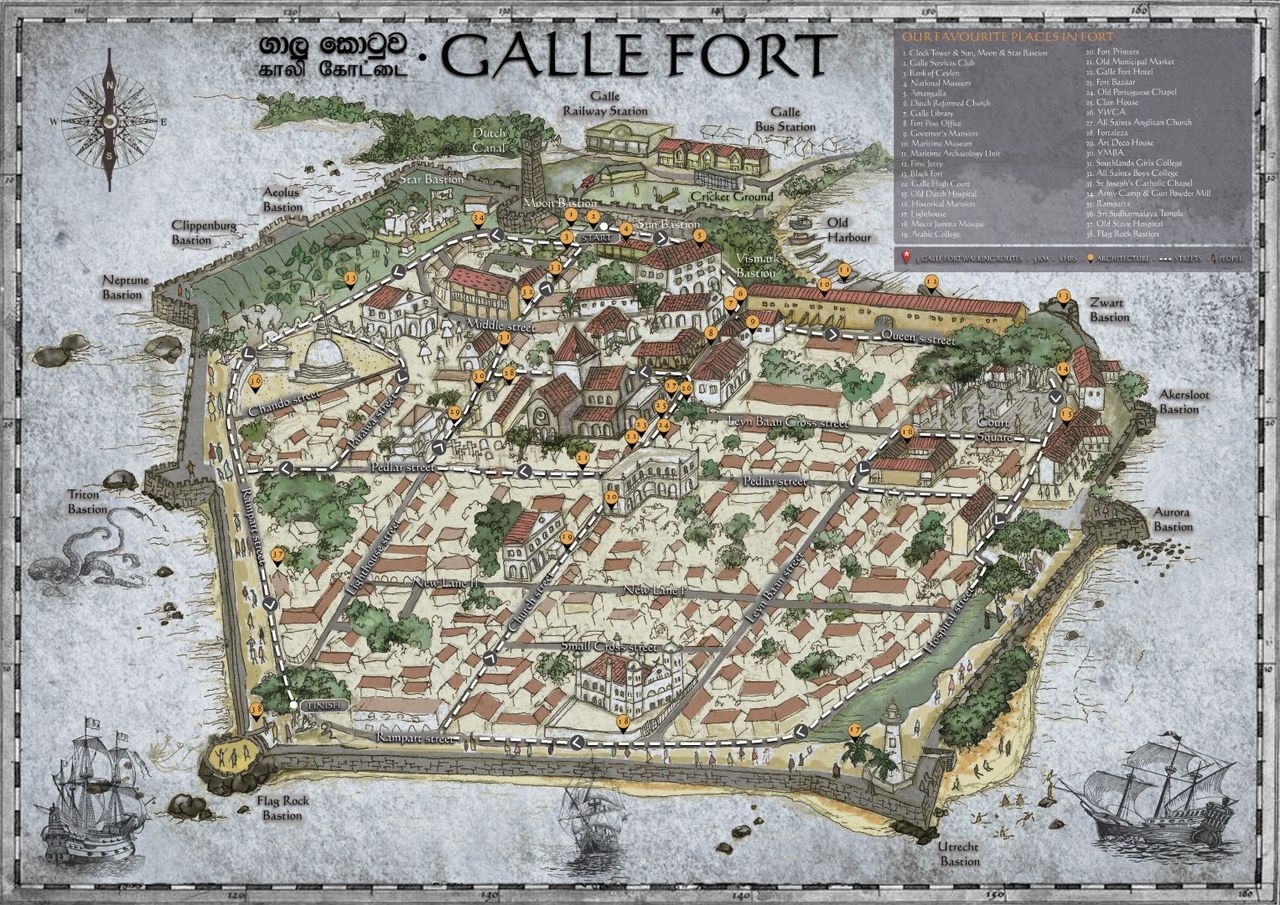This is an intricately detailed fantasy map titled "Galefort" that resembles a city. The map is rectangular, wider than it is tall, and surrounded by a black and white border. At the top left, there is a compass rose, and directly beneath it, a list of different places within the fort is noted, though the text is small and somewhat difficult to read. The top right corner features a key titled "Our Favorite Places in Fort," with numbers corresponding to notable locations marked by small orange circles. 

Galefort itself is depicted as an island, surrounded by blue water and enclosed by a gray brick wall. Within the city boundaries, you can see a collection of densely packed buildings, predominantly with brown rooftops, ranging from large structures to smaller residential ones. The map also depicts some greenery and a few trees dotting the area, though these green spaces are relatively small. The intricate street lines frame the cityscape, adding to the detailed illustration. 

Additionally, several boats, including large sailboats, are shown near the outer edge of the map, emphasizing its island nature. There is some text in a symbolic language on the left side of "Galey Fort," adding to the map's fantasy and artistic elements. The map provides a detailed and imaginative depiction of the city of Galefort, perfect for a game or fantasy setting.